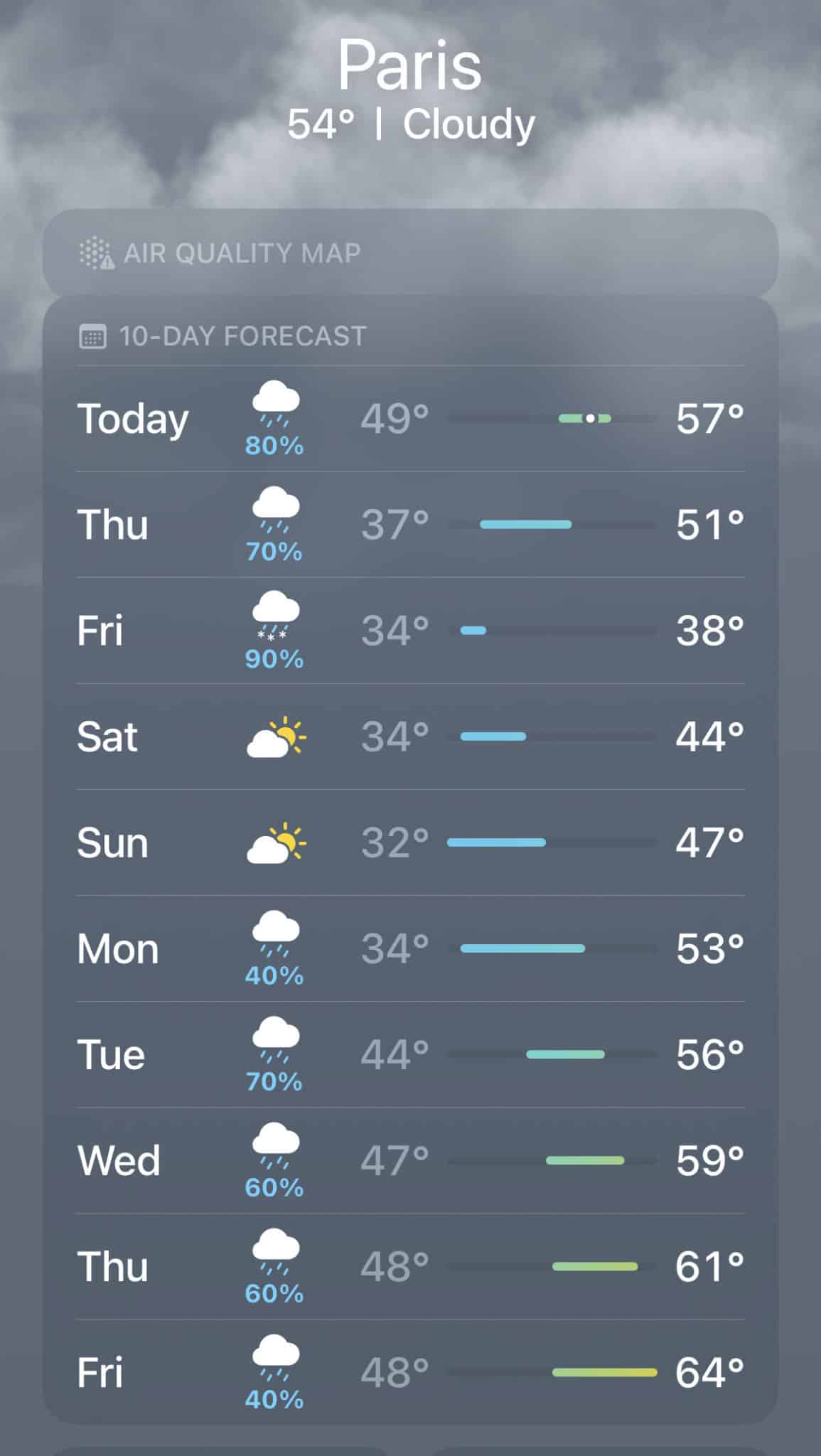A mobile screenshot from a weather app displayed on a cell phone, captured in landscape mode and stretched to enlarge its view. The background features an image of a dark, overcast sky. At the center of the screen, "Paris" is prominently displayed in large white letters, with "54°" shown in large white numbers below it. To the right of the temperature, the word "Cloudy" is written in large white letters. 

At the top of the screenshot, a semi-transparent bar stretches across the screen, labeled "Air Quality Map." Directly beneath this, another equally long bar is labeled "10 Day Forecast." This section displays a vertical list of days, each accompanied by visual rain percentages to the left, icons representing varying weather conditions (clouds, sun), and numerical high and low temperatures for each day. Between the high and low temperatures, a small horizontal bar with different colors and lengths provides a visual representation of the temperature variations throughout the day.